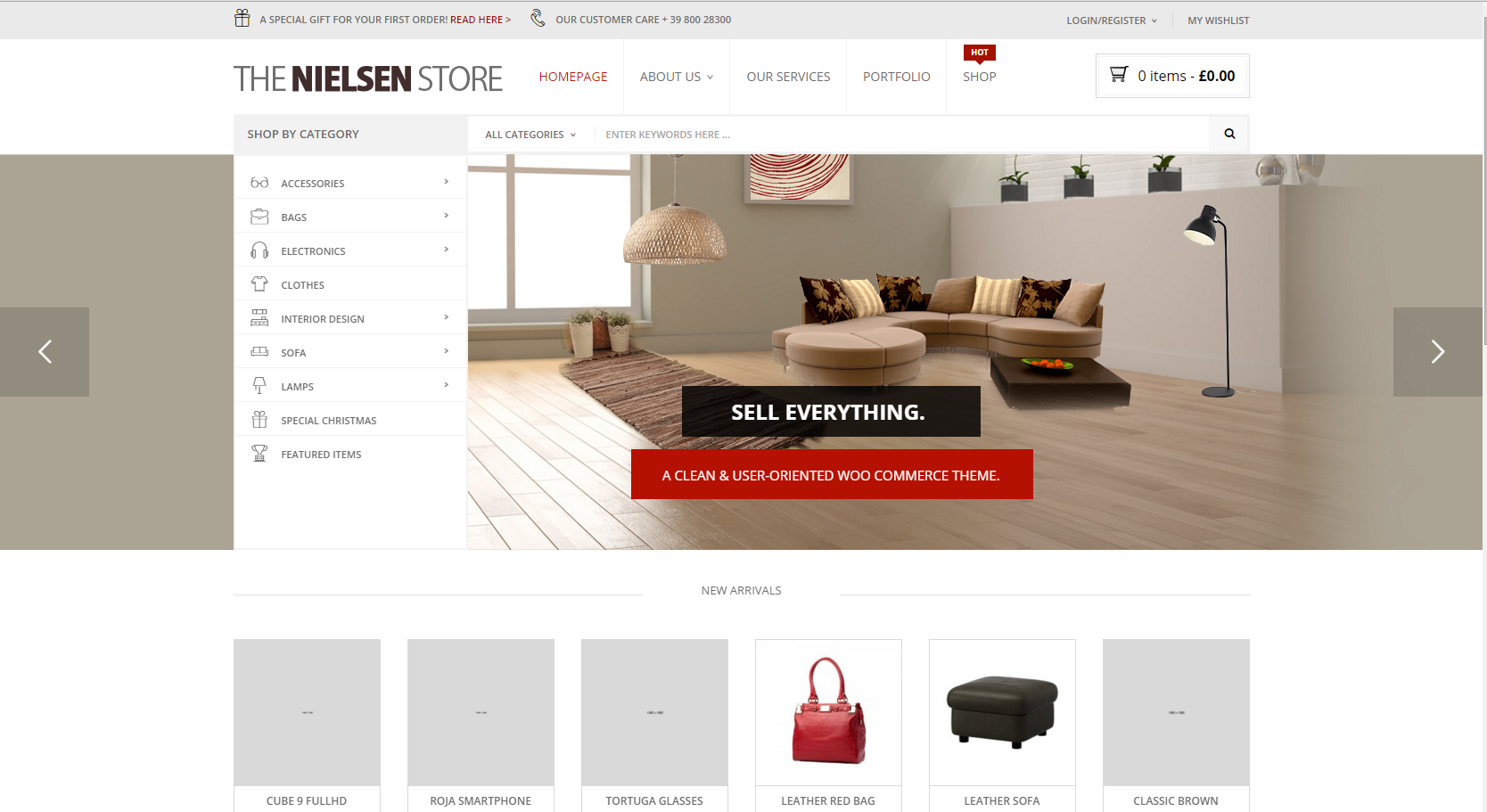The image depicts the homepage of a furniture e-commerce website called the Nielsen Store. The top section of the site features a gray banner with the text "A special gift for your first order" and "Read here" highlighted in red. To the right of this banner, contact information is provided with "Customer Care 3980028300." Further to the right, menu options for "Log In," "Register" accessible via a pull-down menu, and "My Wishlist" are displayed.

Beneath the top section lies a pristine white navigation bar indicating the "Nielsen Store" title alongside menu options: "Home Page" (in red), "About Us" with a dropdown selection, "Our Services," "Portfolio," and "Shop" which has a "hot" label next to it. Additionally, a shopping cart icon shows "Zero items - Zero pounds."

Central to the webpage is a prominent photograph showcasing a stylish living room. The image features a circular couch, a low black table, and beige walls, accentuated with the bold text "Sell everything." This text is displayed on a rectangular strip, and below it, the description "A clean and user-oriented WooCommerce theme" clarifies the purpose of the site as hosting a theme for WooCommerce.

Below the primary image are six smaller boxed sections, four of which are greyed out. The remaining two display a red leather handbag and a black ottoman, indicating the types of products offered by the store.